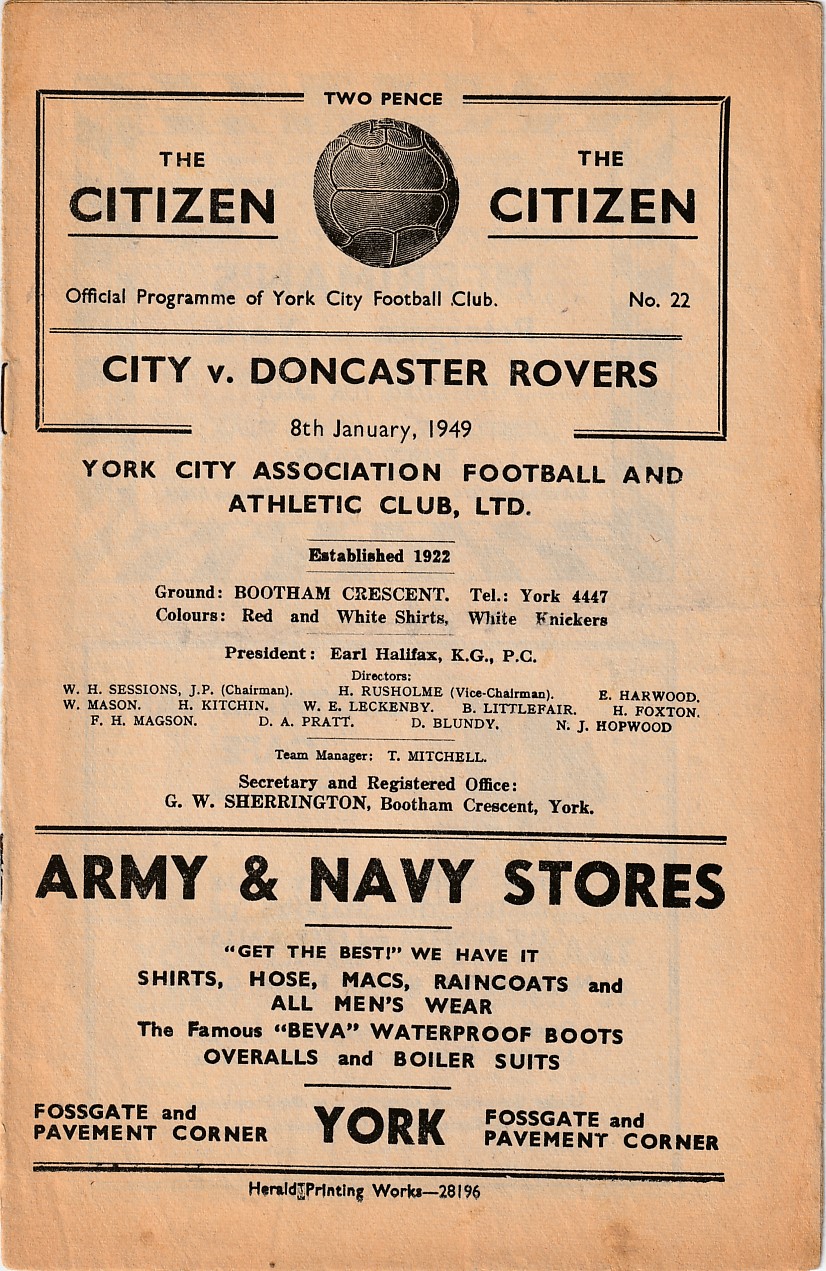This image showcases the cover of "The Citizen," the official program for York City Football Club, priced at 2 pence. The cover prominently features a soccer ball with the title text printed on either side. Below the ball, it details the edition number (No. 22) and lists the match between York City and Doncaster Rovers on January 8th, 1949. The program also notes that York City Association Football and Athletic Club Limited was established in 1922, with their home ground at Bootham Crescent. The club's colors are red and white shirts with white shorts. The president listed is Earl Halifax, KG, PC, along with directors A.W. Sessions, H. Ross Lum, E. Hardwood, W. Mason, H. Kitchen, W.E. Lacking, B. Littlefair, H. Roxton, F.H. Magazine, D.A. Pratt, D.L. Boondi, and N.J. Hopwood. 

An advertisement for Army and Navy Stores highlights their offerings, claiming "Get the Best. We have it." They offer a range of menswear including shirts, hosiery, macs, raincoats, waterproof boots, overalls, and boiler suits. The store locations are noted as Pavement Corner, York, and Fossgate. The cover design is gray on a faded brown background, adding a vintage feel to this historical document from 1949.